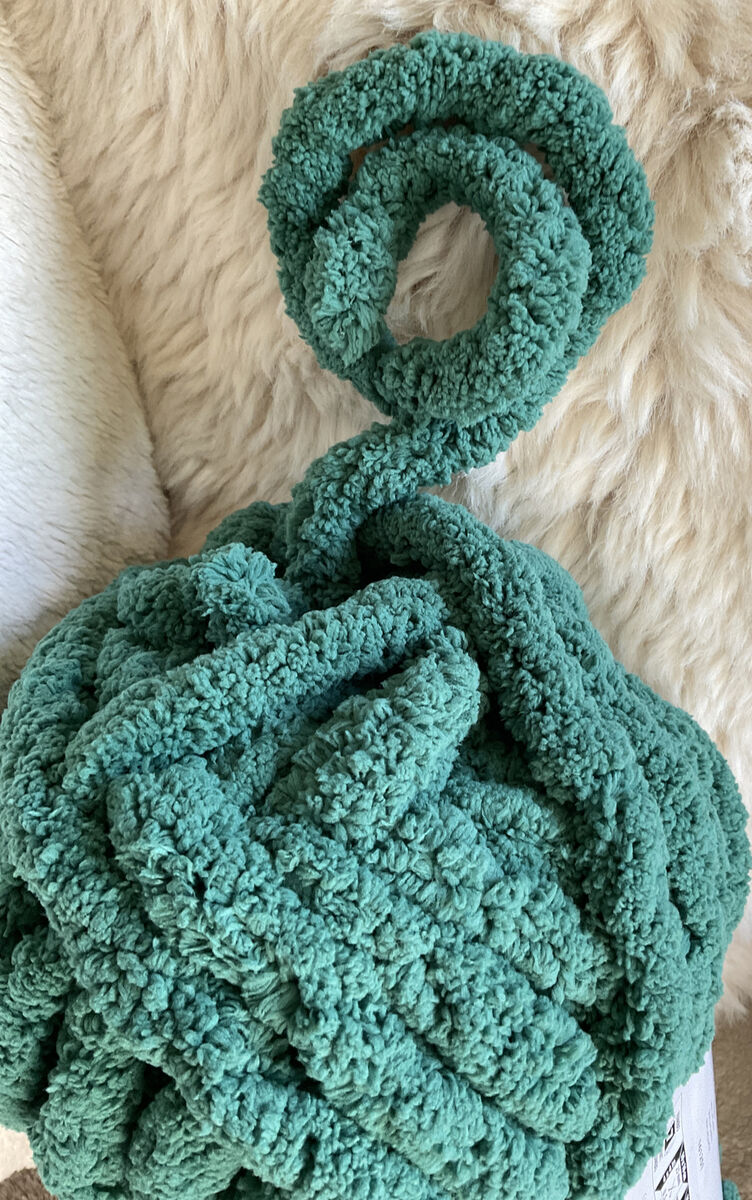This image prominently features a tightly wrapped ball of thick, dark green blanket yarn, positioned near the bottom of the frame. A single strand of the yarn extends from the top of the ball, looping around in a cinnamon roll or antenna-like shape. The background consists of a fuzzy white surface that appears to be either a shag rug or a plush chair, with a visible armrest on the left side suggesting the latter. The yarn ball rests both on this fuzzy surface and on a white box beneath it. Elements of carpet or a wall are faintly visible on either side of the box, framing the scene. The yarn itself appears highly textured, suggesting it could be stretchy or capable of holding shapes, and displays varying shades of green, contributing to its dynamic and cozy appearance.